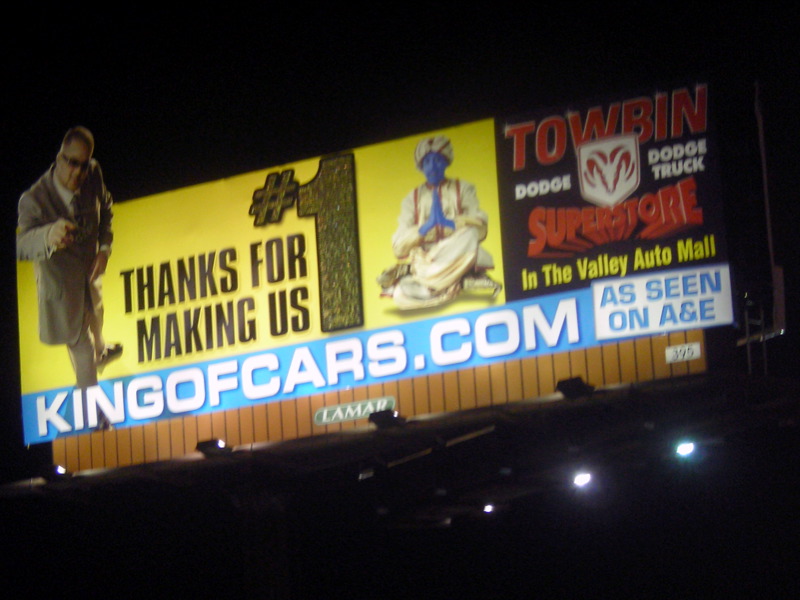This color photograph, taken at night, prominently features a large illuminated billboard. The billboard's design is primarily yellow with a black section on the right and a blue banner at the bottom. On the left edge, a photo of a man in a dark brown suit is displayed. He has short hair and is wearing sunglasses. Next to his image, a triumphant message reads, "Thanks for making us number one." Adjacent to the message is a figure dressed as a genie, complete with a turban and a long, flowing caftan. The genie, with their face and hands painted blue, is seated cross-legged in a prayerful pose, adding a whimsical touch to the advertisement. To the far right, within a black square, is the text "Tobin T-O-W-B-I-N Dodge" and "Dodge Truck," accompanied by the Dodge logo and the words "Superstore in the Valley Auto Mall." Below this, a blue banner at the bottom of the billboard reads "kingofcars.com as seen on A&E," promoting an associated online presence and television feature.